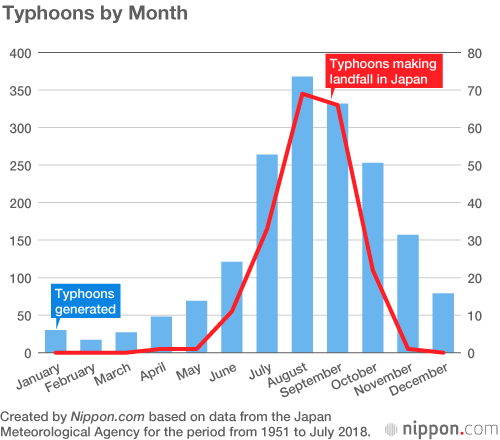The image is a detailed bar graph titled "Typhoons by Month," created by Nippon.com based on data from the Japan Meteorological Agency for the period from 1951 to July 2018. The graph features blue bars labeled "Typhoons Generated" and a red line labeled "Typhoons Making Landfall in Japan." The left y-axis ranges from 0 to 400, indicating the number of typhoons generated, while the right y-axis ranges from 0 to 80, representing the number of typhoons making landfall. The x-axis displays the months from January to December. The background is white, and both axes are clearly marked. The data shows that typhoon activity is highest between July and October, with the peak occurring in August, where both the tallest bar and the highest point of the red line are observed.